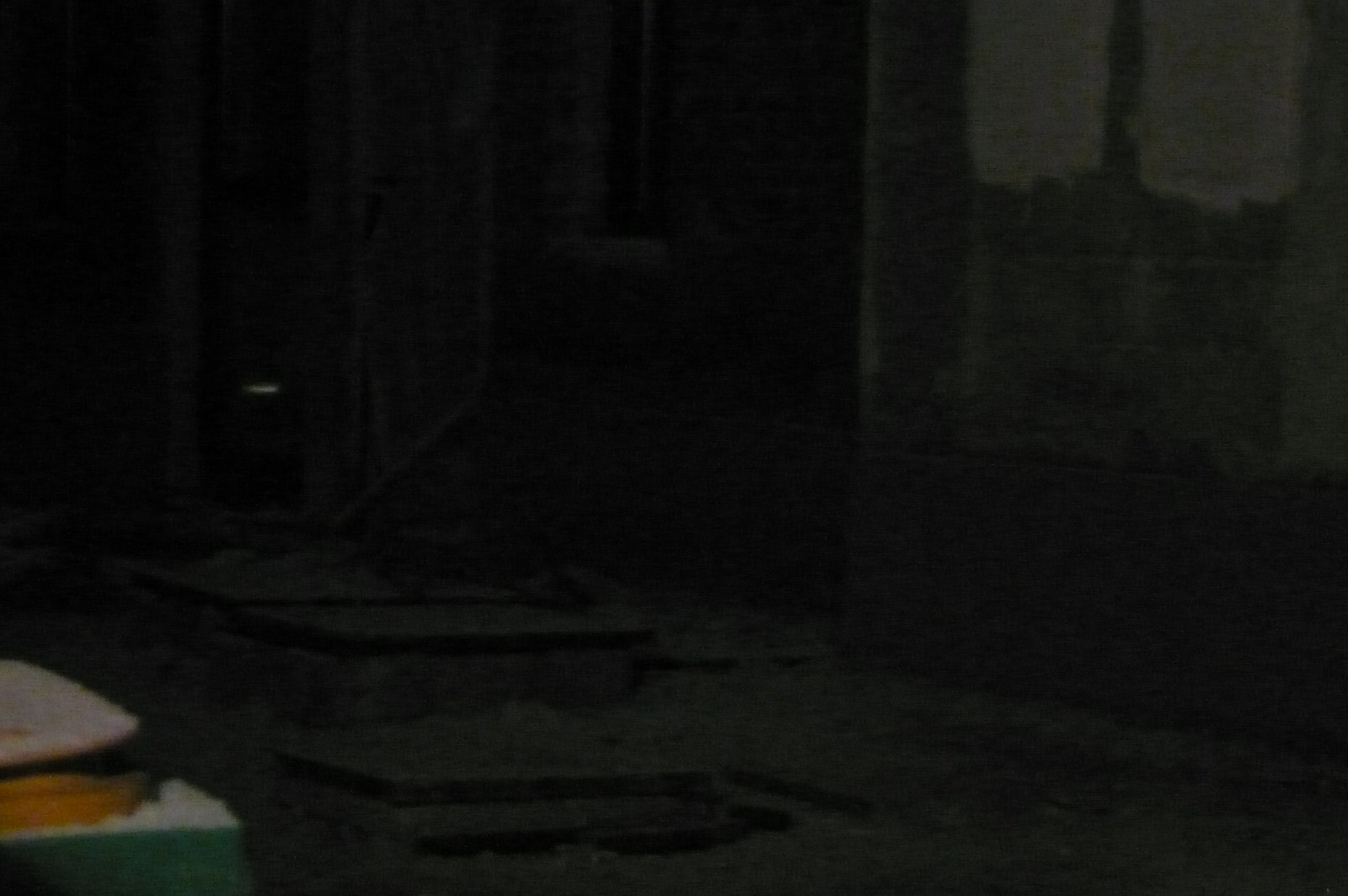This photo, taken at night and of notably low quality, presents a challenging scene to decipher. The image appears to be captured outdoors after a snowstorm, with snow prominently covering the ground. On the bottom left corner, there's an indistinct object that might be a pair of trash bins, barely visible. The scene gives the impression of an abandoned or deserted area. To the right, you can see a concrete or brick wall with two distinct, white painted patches at the top. The left side suggests a possible stair pattern or steps leading up, and there might be a faint reflection of a car light. In the very center, there's an element that could be a door, seemingly open, with a hint of a rug on the floor and a coffee table with something on it. The colors faintly observable in the scene include yellow, white, and green. Overall, the photo heavily emphasizes an eerie, desolate atmosphere underpinned by the difficult-to-decipher details in the dim light.